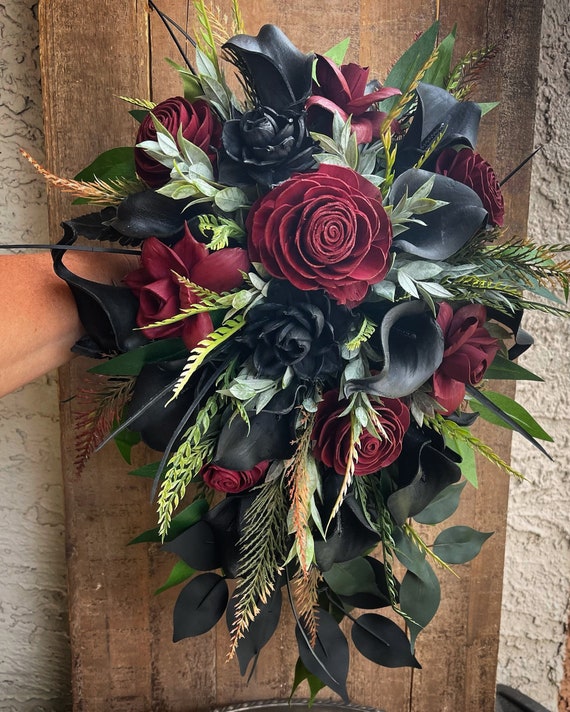In the photograph, a floral arrangement is held up against a wooden plank that leans against a textured cement or stucco wall. The bouquet, consisting of deep maroon flowers, black dyed flowers, black leaves, and evergreen foliage, is being positioned by a partially visible arm extending into the frame. The background includes gray chairs beneath the arrangement, adding context to the setting. Despite the dramatic colors of the flowers, which lend a somber yet striking aesthetic, the overall composition captures a moment of quiet beauty and intention.